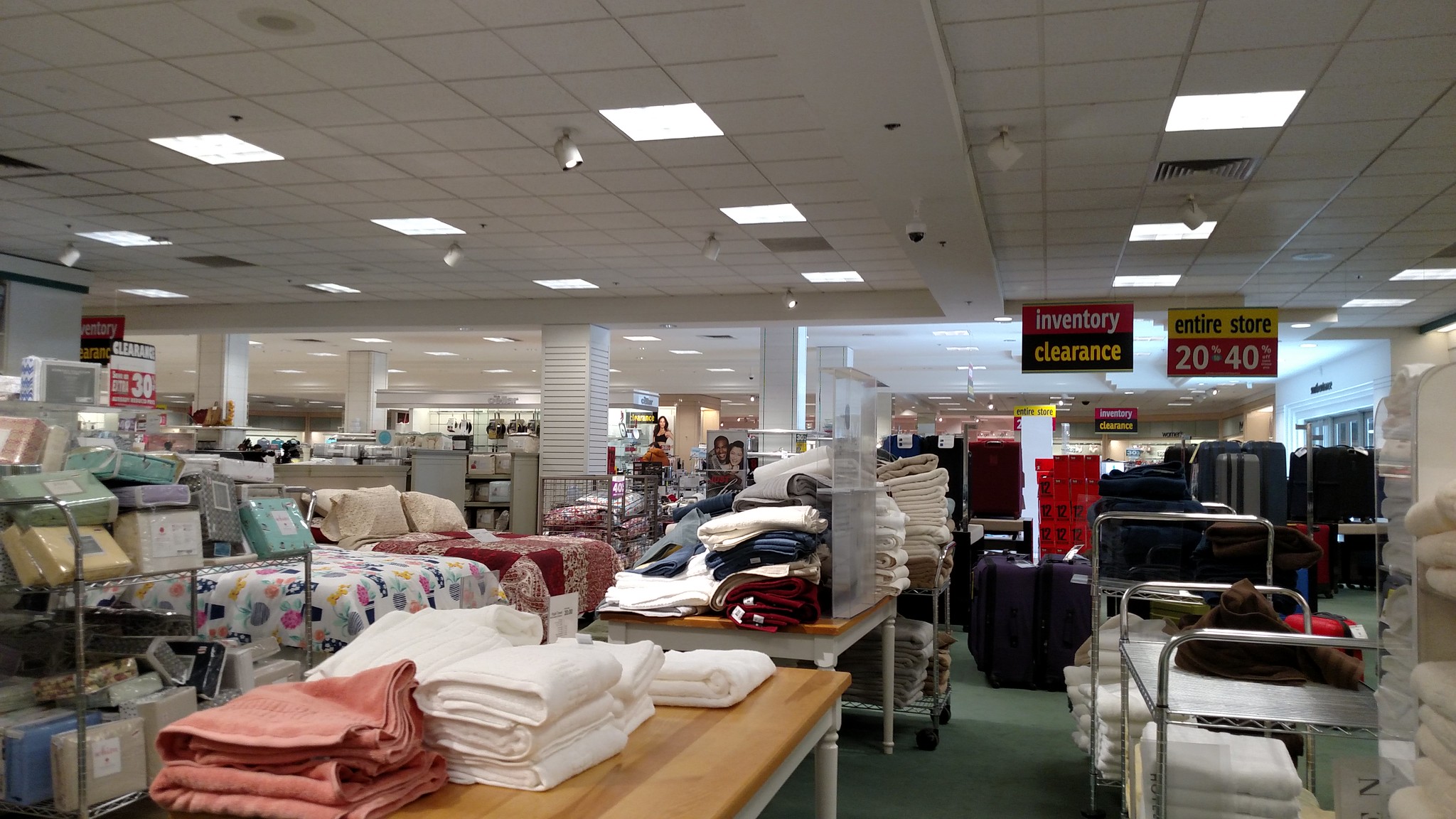The image depicts a bustling retail store specializing in bedding and towels, currently having an inventory clearance sale. The store is filled with various bedding items, including beds dressed with comforters and pillows, all neatly arranged. Shelves hold additional pillows, while multiple tables display neatly folded towels and bedding.

The floor of the store is covered with green carpet, and there are metal racks to the left laden with an assortment of pillows. The pillows come in various colors such as yellow, green, cayenne, light green, and mint. The towels, organized by color, include white, pink, orange, brown, red, and blue options.

Prominent signs throughout the store announce significant discounts, with entire store sections marked at 20% and 40% off, indicating this is the clearance section. There are hints of other signs in the background, possibly also advertising the clearance sale with "Edmunds Clearance" text. Overall, the image captures the extensive variety and bustling atmosphere of a retail store in the midst of a major clearance event.